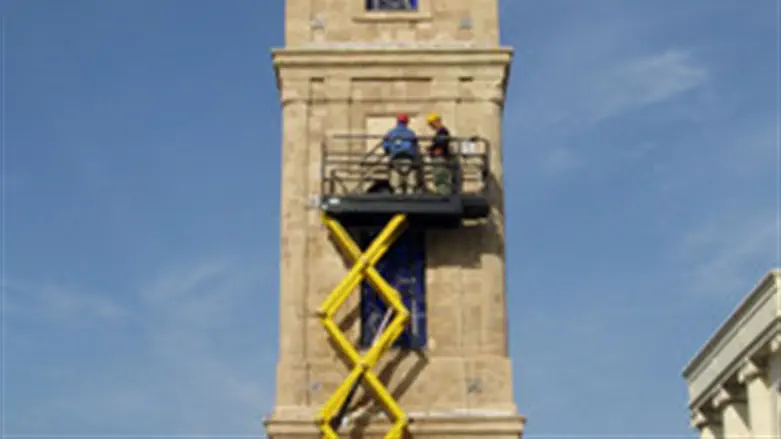The image captures an outdoor scene featuring two men atop a tall beige-colored tower with big, closed windows, appearing to be involved in repair work. They are standing on a yellow elevating crane with a black top and railings, positioned against the building. The man in the center is dressed in a blue shirt and a red hard hat, while the one next to him wears a black shirt and a yellow hard hat. In the background, the sky is a clear blue with a few wisps of white clouds, suggesting a sunny day. To the right, partially visible, is another monument-like structure with white columns. The photo is slightly blurry and taken from a lower angle, emphasizing the height of the tower and the crane as it extends down below them.